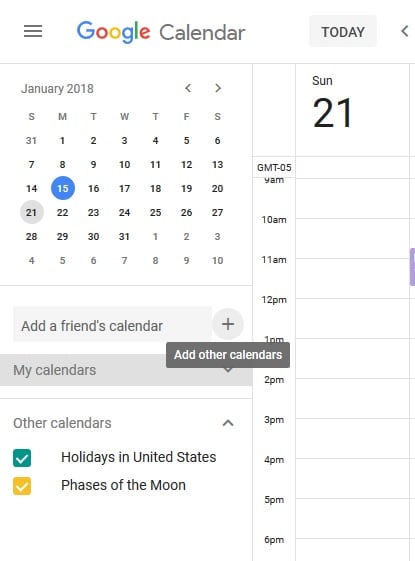The image displays a Google Calendar interface for January 2018. A blue circle highlights January 15, while January 21 is marked with a gray circle. Below the calendar, a gray circular button featuring a plus sign accompanies the text "Add a Friend's Calendar." The interface includes sections labeled "My Calendars," "Other Calendars," "Holidays in the United States," and "Phases of the Moon." On the right side, details for Sunday, January 21 are shown, with time slots ranging from 9 a.m. to 6 p.m., each within a designated box. A small purple tab is also visible on the right. The top right corner displays a left arrow, and the top left features an icon with three black or gray lines. The Google logo, in its signature blue, red, yellow, and green colors, is positioned prominently at the top.